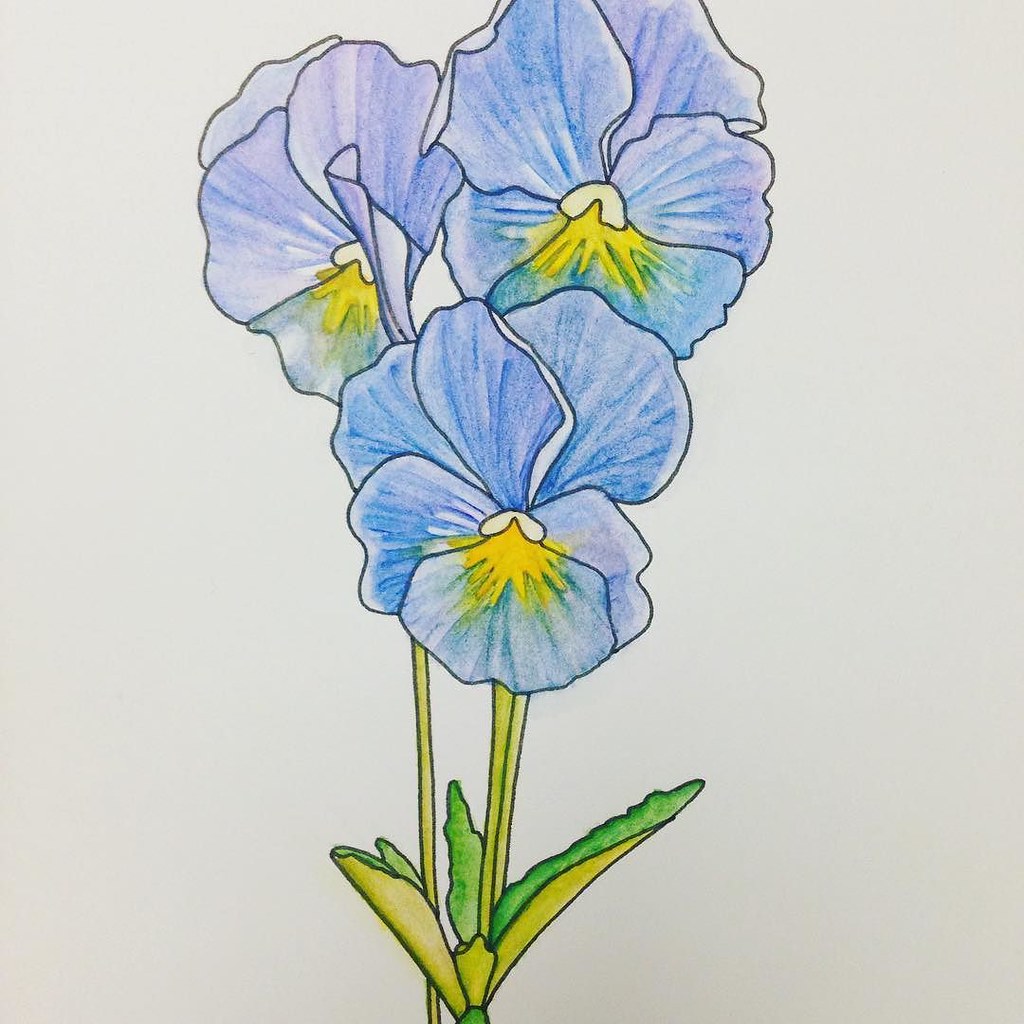This detailed illustration showcases a trio of blue flowers prominently arranged against a solid white background. The flower petals are predominantly blue, with hints of purple and varying in shape, giving a soft and fluffy appearance. Each flower features a yellow center, with a distinctive white, bean-like shape inside it, resembling a piece of macaroni. The flowers are connected by green stems adorned with a few green leaves at the base. The thick and solid line work, paired with what appears to be fine shading done possibly with colored pencils, highlights the intricate details and careful coloring of the artwork. The flowers are bunched closely together, with two flowers positioned above and one shorter flower in the front, creating a cohesive and visually appealing composition.